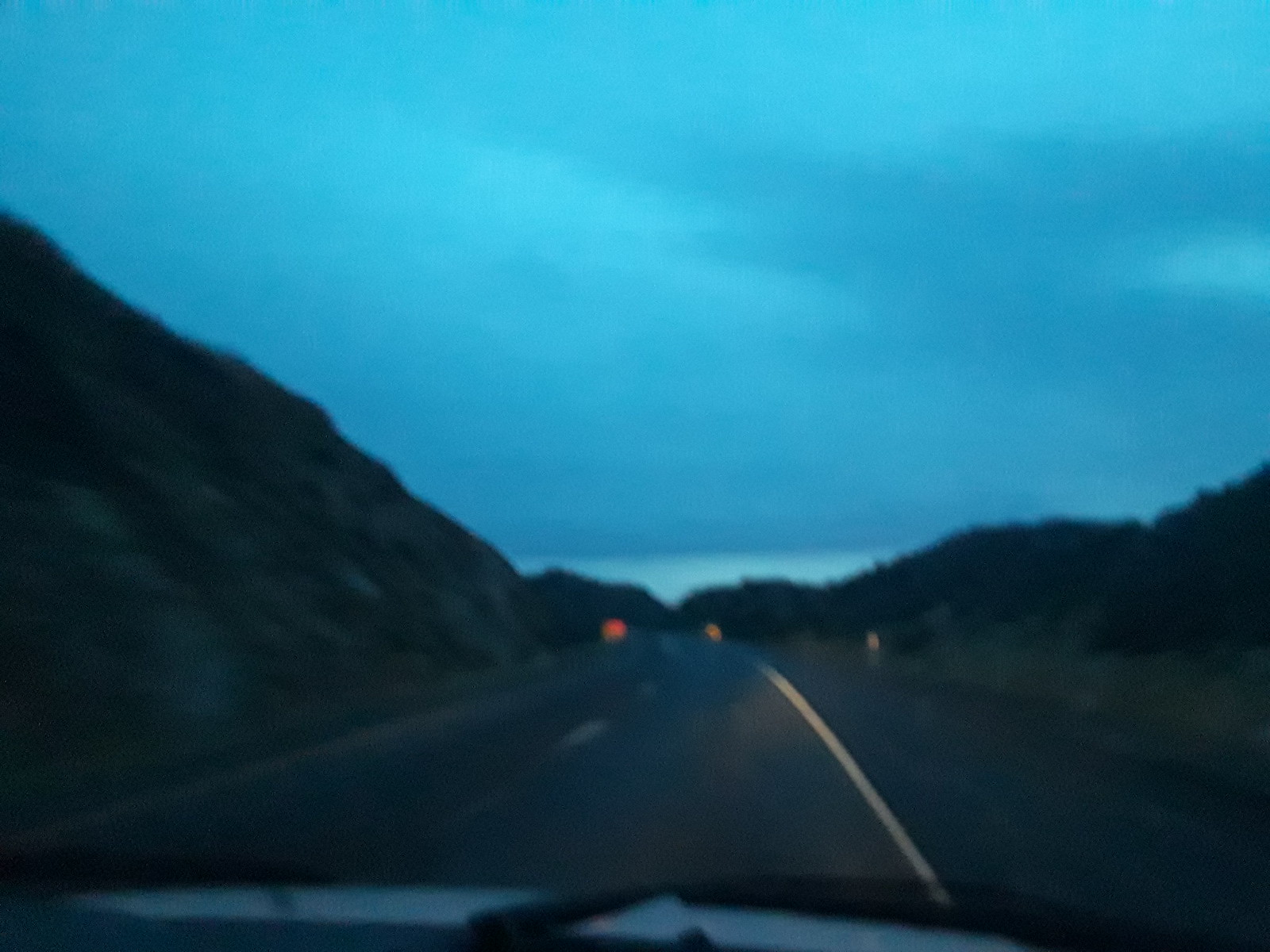A blurred photograph captures a twilight scene of a hilly road, taken from the dashboard of a moving vehicle. The darkened foreground and the obscured details impart an almost ethereal quality to the image. The background reveals a darkening, yet still faintly light blue sky adorned with scattered clouds. The road itself winds through hilly terrain, with the right side marked by a yellow line that becomes more visible due to the vehicle's headlights. The headlights create a subtle glow, slightly illuminating the yellow line on the right side of the road. A couple of blurry lights are visible ahead, adding depth and mystery to the scene, indicative of distant vehicles or other points of illumination.